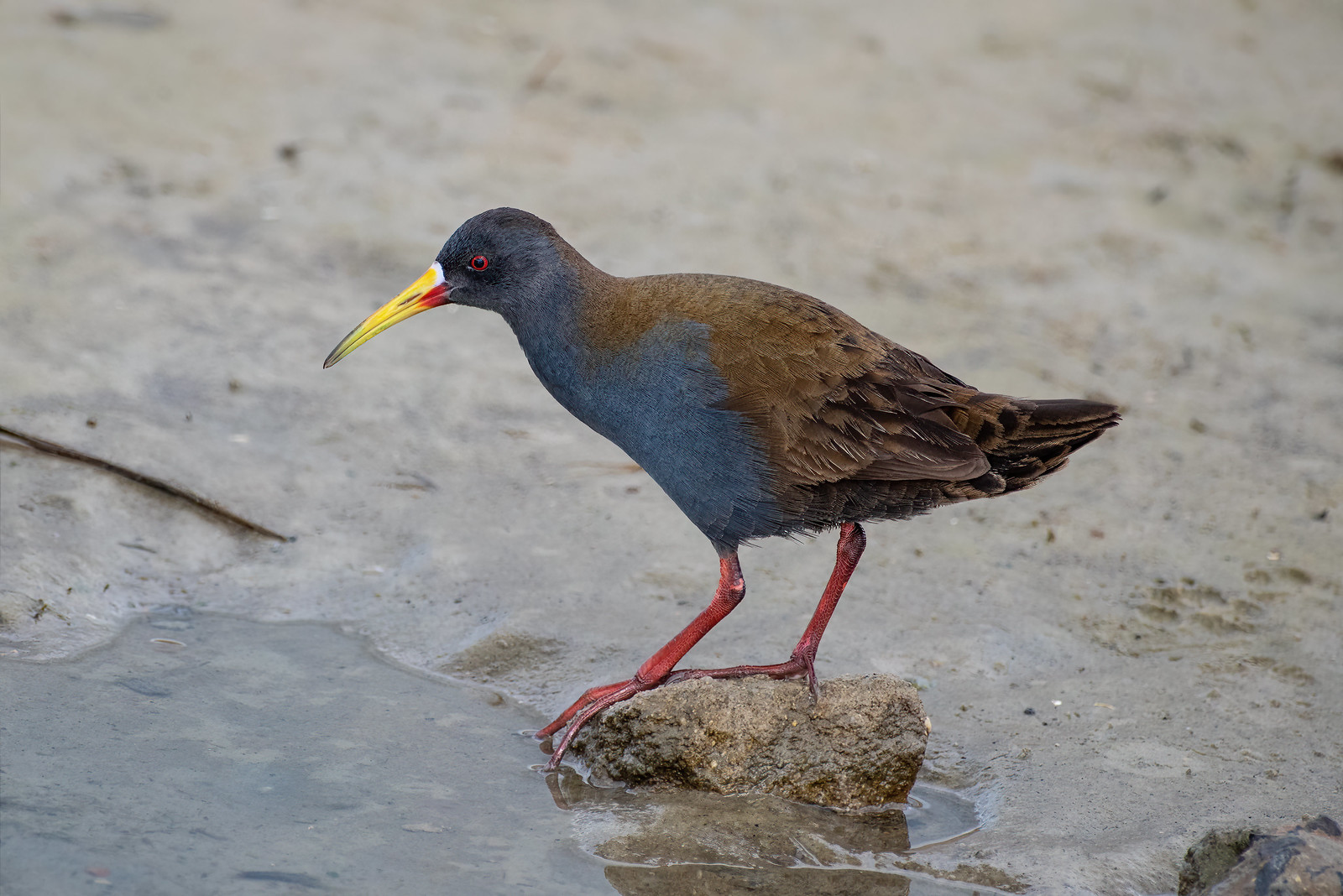In this detailed photograph, a vibrant bird is prominently perched on a tan-colored rock in icy water. The bird, adorned with elaborate colors, features dark blue and brown feathers, a strikingly yellow beak with red and green at its base, and vivid red legs. Its eyes are red and it has an intense gaze. The bird is positioned facing left, seemingly contemplating whether to venture onto the ice that is beginning to crack beneath it. Surrounding the scene, there is more ice and scattered rocks and sticks visible in the background, set against a setting that appears to be a chilly, possibly frozen, body of water. The environment looks wild and natural, captured in a moment of quiet, cold beauty, with the bird standing still and observant.